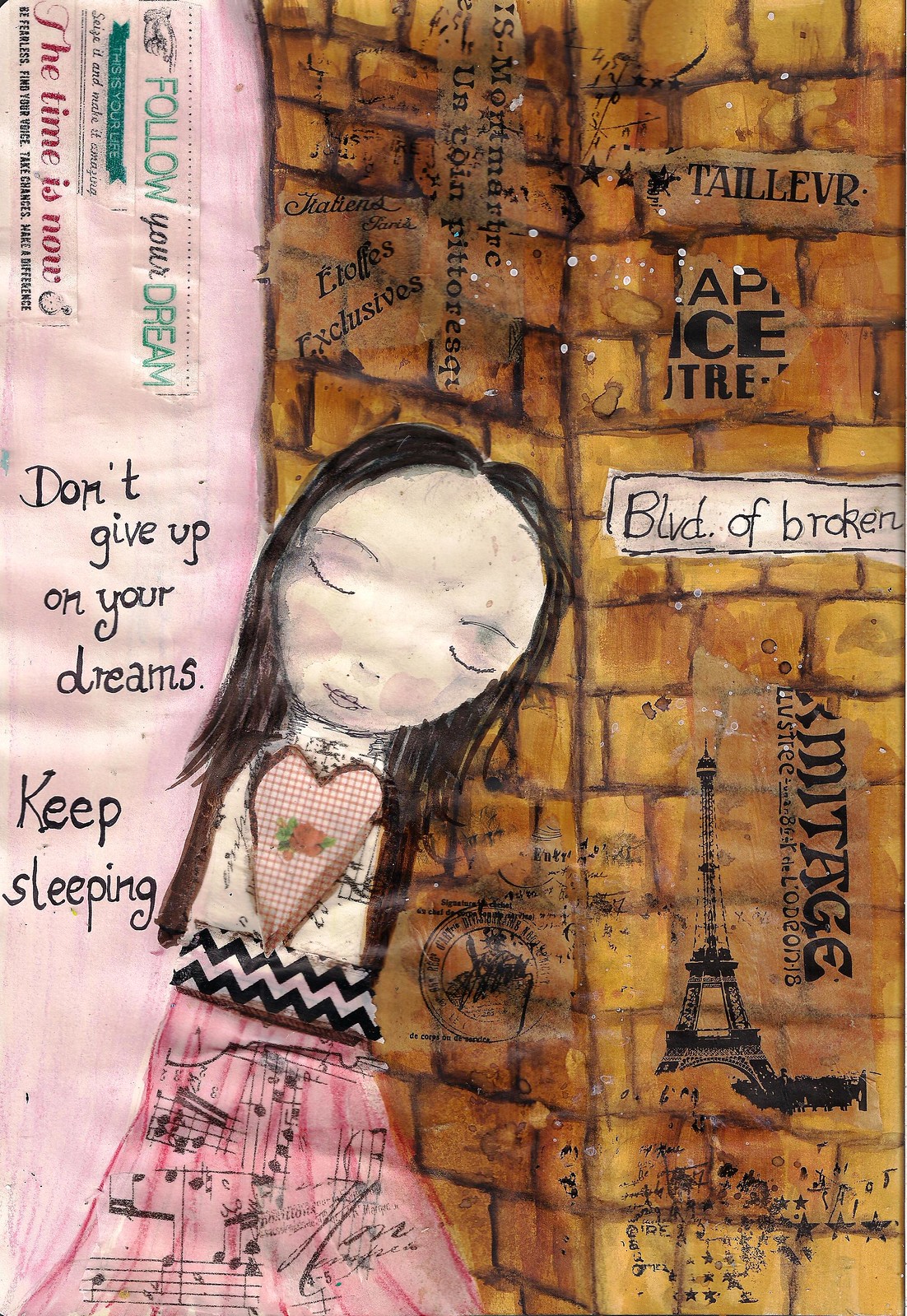The image appears to be a detailed illustration, possibly intended as artwork for a book cover or a poster. Dominating the left side of the rectangular image is a pink vertical banner featuring motivational phrases such as "Follow Your Dreams" and "The Time is Now." Below these, another phrase reads, "Don't give up on your dreams, keep sleeping," stamped across the top of the banner.

In the middle section, a forlorn-looking girl with an egg-shaped head and straight black hair is depicted. Her eyes are merely lines, suggesting that they are either closed or she's looking down, contributing to her sad demeanor. The girl is wearing a white and black zigzag-patterned waistline and a pink skirt adorned with musical notes. Her t-shirt has a heart on it, which looks as if it is sewn onto the fabric.

She stands against a yellow brick wall that turns a corner, creating an artistic complexity within the illustration. Various words are scattered across the wall, with some intentionally broken or cut off, suggesting fragmentation. Prominently, there is a depiction of the Eiffel Tower illustrated in black on the wall. One of the phrases visible on the wall is "Boulevard of Broken Dreams," reinforcing themes of aspiration and melancholy.

Overall, the image blends elements of aspiration and whimsy with an underlying theme of perseverance amidst challenges.